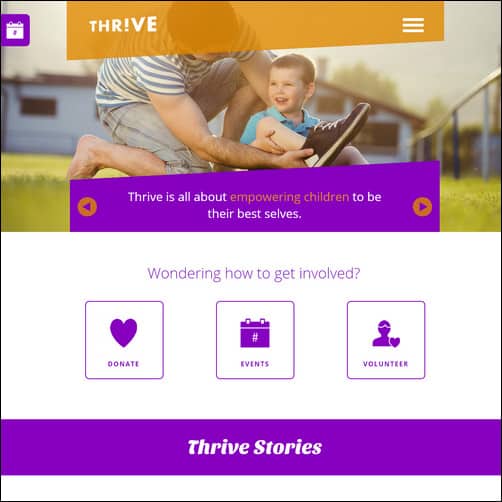This screenshot captures a Thrive (stylized as Thr!ve) web page, marked by an orange banner at the top with the organization’s name, featuring an exclamation mark instead of the letter 'I.' To the right of this banner is a hamburger menu icon. Below the banner, there's a heartwarming photograph of a man kneeling as a child assists him in putting on his shoes, illustrating a moment of connection and support.

Beneath the photo, there is a purple banner with white text that reads, "Thrive is all about empowering children to be their best selves." The phrase "empowering children" stands out in orange text. This banner features navigation arrows on either side, suggesting the ability to browse through additional images or messages.

Following this section, there's a white rectangle with purple text posing the question, "Wondering how to get involved?" Directly below are three purple-outlined boxes, each signifying different ways to contribute. The first box, labeled "Donate," is accompanied by a heart icon. The second box, "Events," includes a calendar icon. The third box, "Volunteer," is highlighted by a torso icon with a small heart.

At the very bottom of the page is another purple banner with white text, announcing "Thrive Stories," likely linking to inspirational narratives related to the organization's mission.